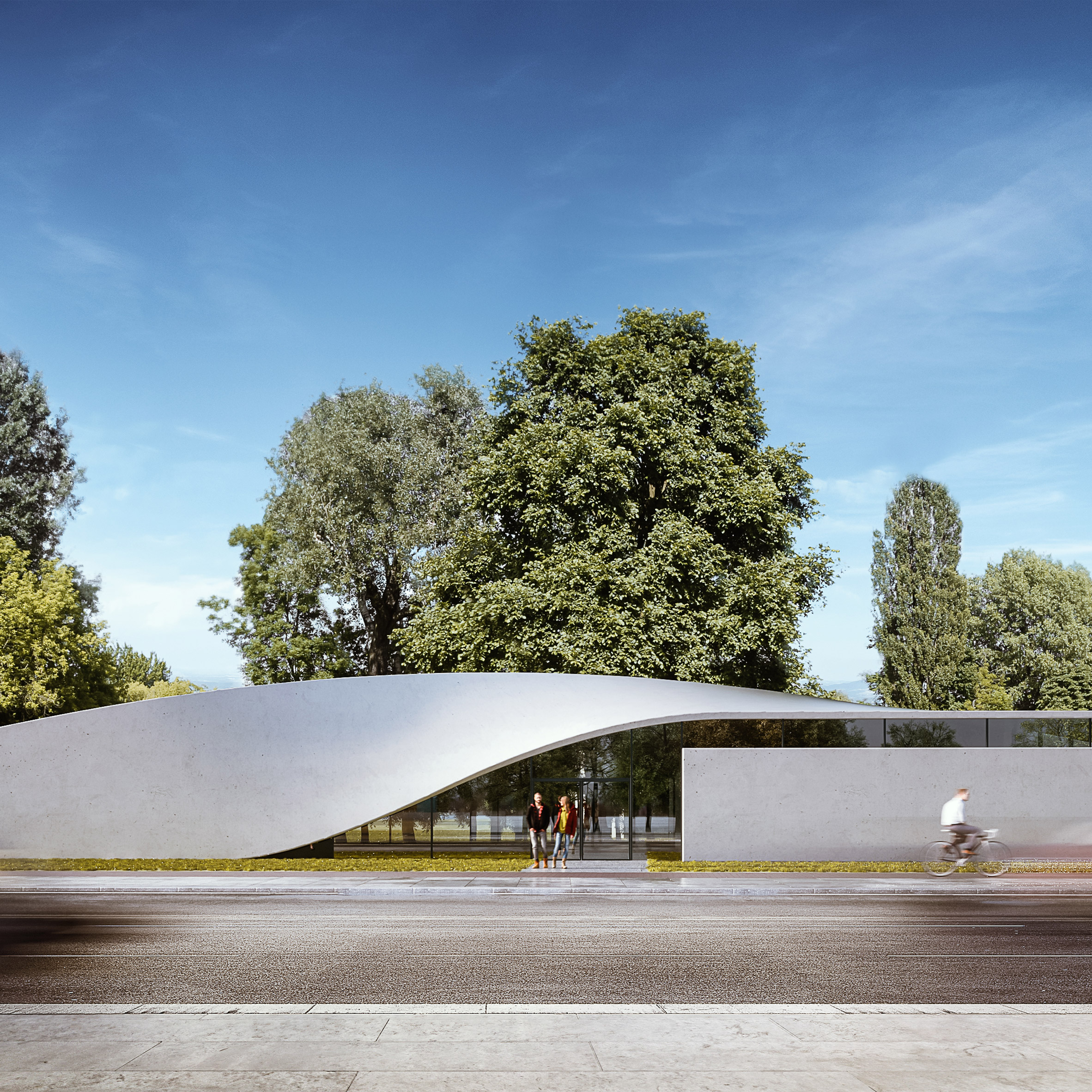In this detailed photograph, taken outdoors during the daytime, we see a vibrant scene featuring a deep blue sky that transitions to light blue near the horizon, adorned with wispy white clouds. Dominating the upper portion of the image is a lush array of green-leafed trees scattered throughout the area, creating a serene and natural backdrop.

Central to the image stands a distinctive gray building with a unique ribbon-like silver roof. This roof unfurls dramatically from the lower left to the center of the picture, creating an eye-catching architectural feature. The left part of the roof touches the ground, while the middle portion arches gracefully overhead at a height of about 15 to 20 feet, before extending rightward.

Underneath this ribbon roof, we see two men wearing blue jeans and jackets, with one notably sporting yellow boots. They walk along a gray asphalt road that occupies a significant portion of the lower image, adding to the structured layout of the scene. Adjacent to this road is a light gray sidewalk, where a person on a bicycle is riding calmly from left to right, with the silver wall of the building as their backdrop.

Altogether, this image captures a picturesque and dynamic outdoors setting, combining natural beauty with striking architectural design and human activity.